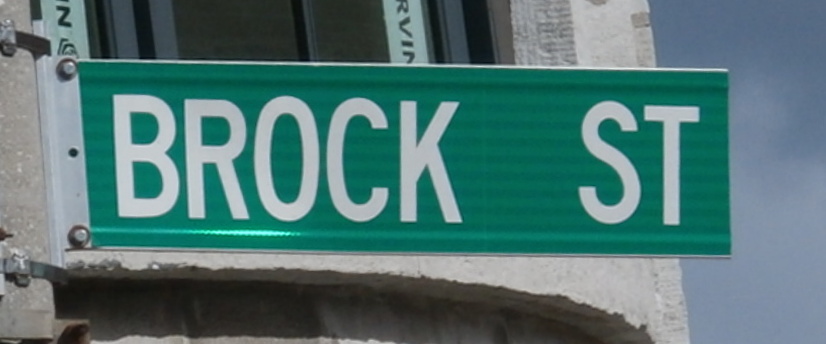This detailed close-up photograph captures a green street sign with "Brock St" written in large, white letters. The sign is mounted with silver bolts onto a white metal bracket. The background appears to be a building with a gray cement facade and a black window at its center, though the exact structure remains indeterminate. To the right of the sign, a patch of blue sky with wispy clouds is visible, adding a touch of color contrast to the scene.